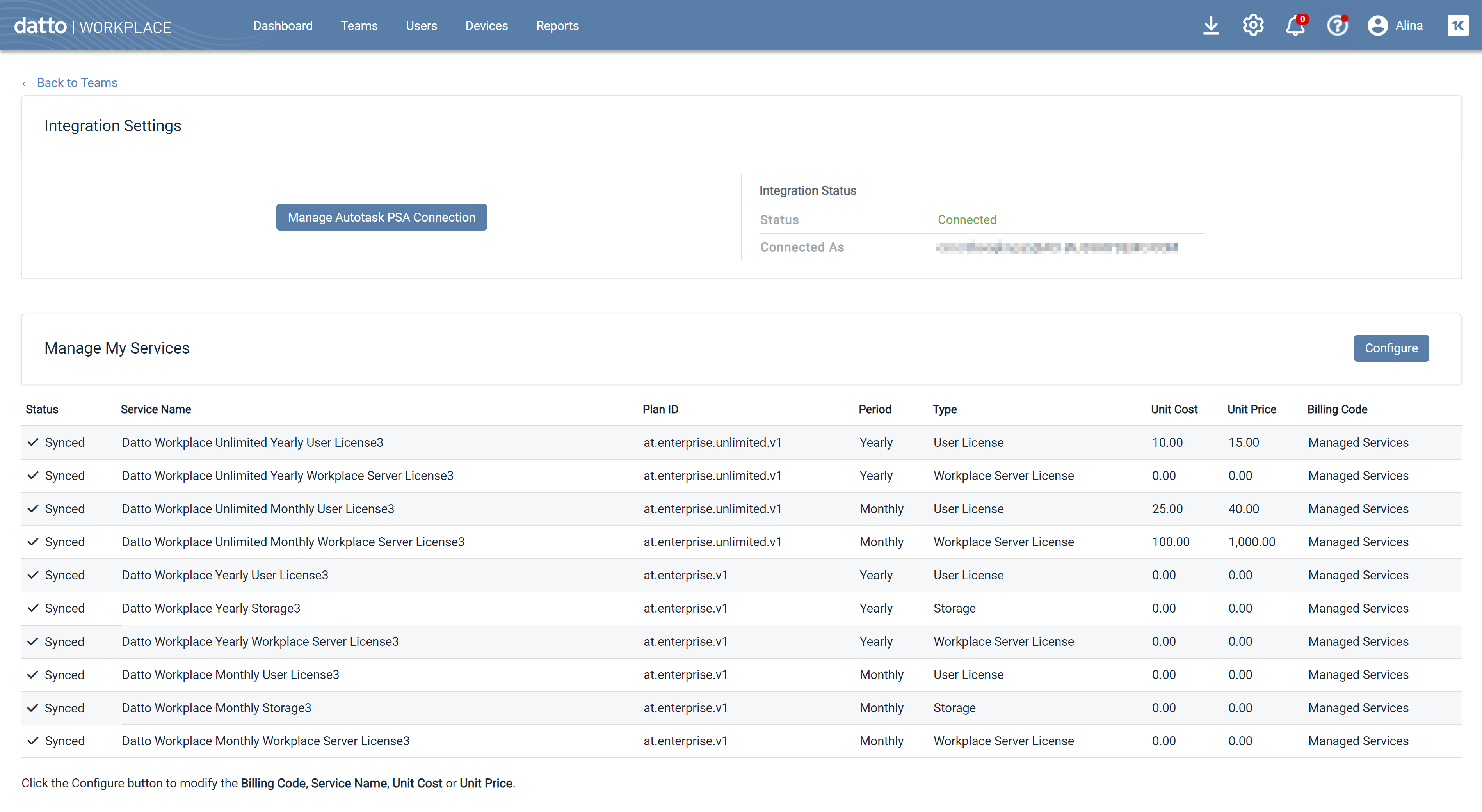The image depicts a page from Datto Workplace, a cloud-based service platform. The interface appears to be busy, with multiple settings and navigation options visible, albeit in small, hard-to-read fonts. At the top of the page, there are several main navigation links, including Dashboard, Teams, Users, Devices, and Reports. To the right, additional links are available, including a Download button, Settings, Notifications, and Help.

The user currently signed in has a name starting with "A," possibly "IARA," though the rest of the name is unclear. There are some unread notifications indicated by a dot hovering over the Help button, the nature of which is uncertain whether it was added through editing software or part of the UI.

The main section of the page is aligned with various settings, specifically integration settings, with options like Manage, Auto, Task, and Connection. Further down, there is a section titled "Manage My Services," which lists various Datto Workplace services. Items in this list include "Datto Workplace Yearly," "Datto Workplace Unlimited," and others, whose specific purposes are not detailed in the image.

Overall, the page seems to be a centralized hub for managing different aspects of Datto Workplace services with options for detailed configurations and settings.